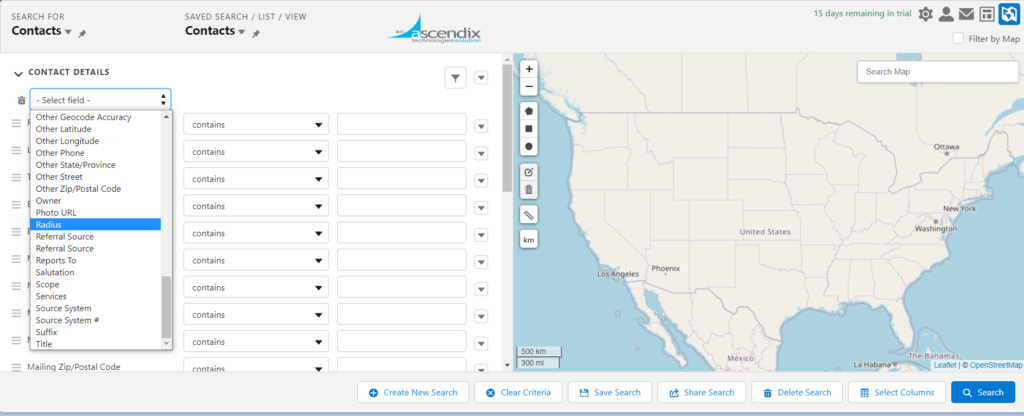The screenshot appears to be of a web interface from Ascendix Technologies. The interface is a contact management tool, featuring a complex and detailed layout.

The webpage is predominantly categorized into various sections for efficiently searching and managing contacts. Measures approximately 10 inches wide by 3.5 inches tall, the interface begins with a header that contains a search bar labeled "Search for Contacts" and several navigation options including "Save Search" and "List View."

On the left-hand side, there is a menu allowing users to specify contact details through various fields such as radius, street, postal code, and owner. Currently, the menu is expanded, covering additional options that are likely underneath. Adjacent to this menu is a column labeled "Contains," featuring dropdown arrows for further selections. Another column allows for manual input, and yet another box with a dropdown arrow provides more selection options.

A map of North America, specifically indicating areas within the United States, Canada, and Mexico, is featured prominently. On this map, major cities like Los Angeles, Phoenix, Washington, New York, and Ottawa are marked, likely indicating locations where Ascendix has centers.

The top of the page displays a notification about "15 days remaining in trial," accompanied by various symbols for settings and personalization options. Users can also filter or search on the map. At the bottom of the page, there are options to "Create New Searches," "Clear Criteria," "Save Search," "Share Search," "Delete Search," and "Select Columns," granting users comprehensive control over their searches and contact management.

Overall, the interface is robust, providing a wealth of features designed to facilitate detailed and efficient contact management within the Ascendix platform.